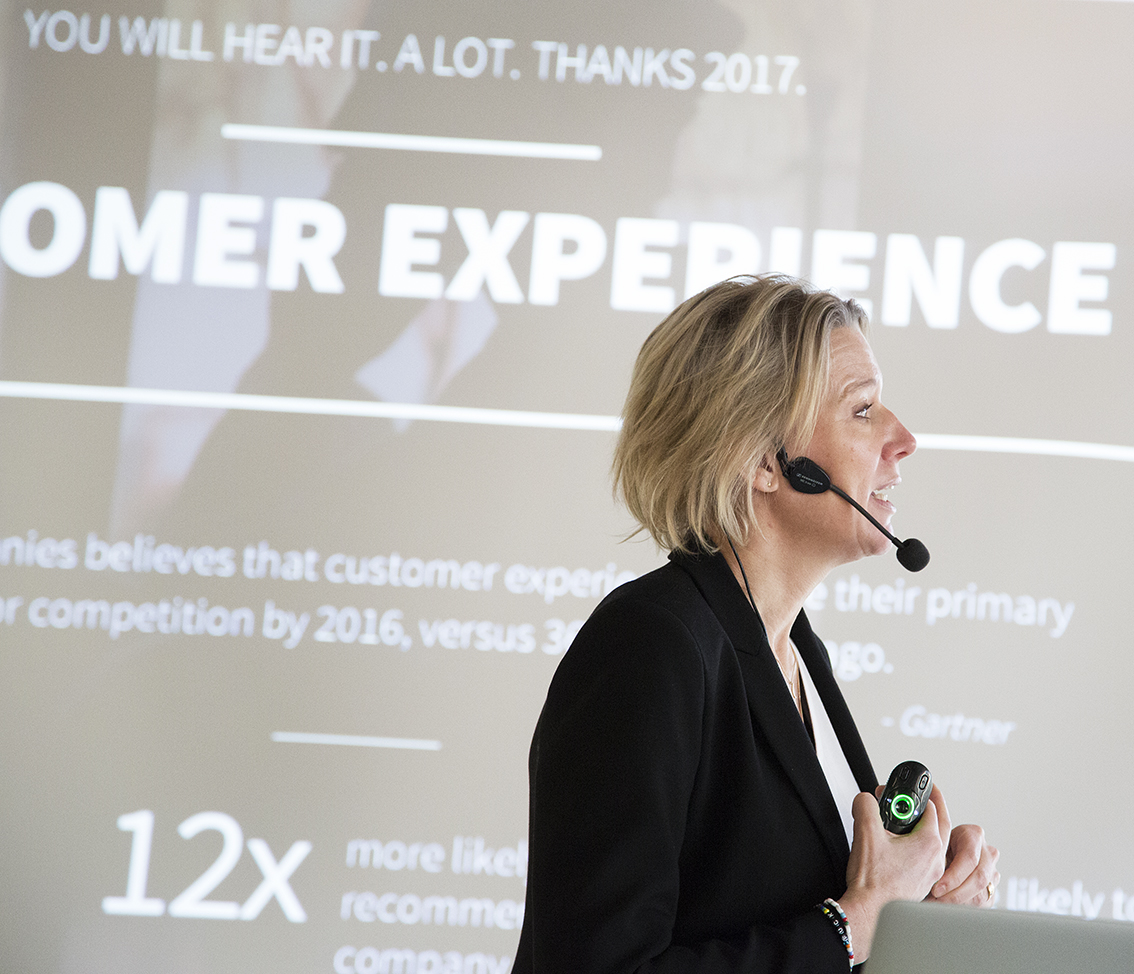The photograph features a blonde woman with shoulder-length hair, captured in a side profile as she delivers a presentation or lecture. She is dressed in a black formal blazer layered over a white shirt. A black over-the-ear microphone is strapped to her right ear, curving around toward her mouth, and she holds a presentation clicker, identifiable by a small green LED light, in her hand. Positioned centrally in the image, she appears to be facing an audience, possibly at a conference. Behind her is a projection screen with white text, partially readable and referring to customer experience and competition, including phrases like "You will hear it a lot. Thanks, 2017." Additionally, there is a grey laptop in front of her, reinforcing the context of her presentation.